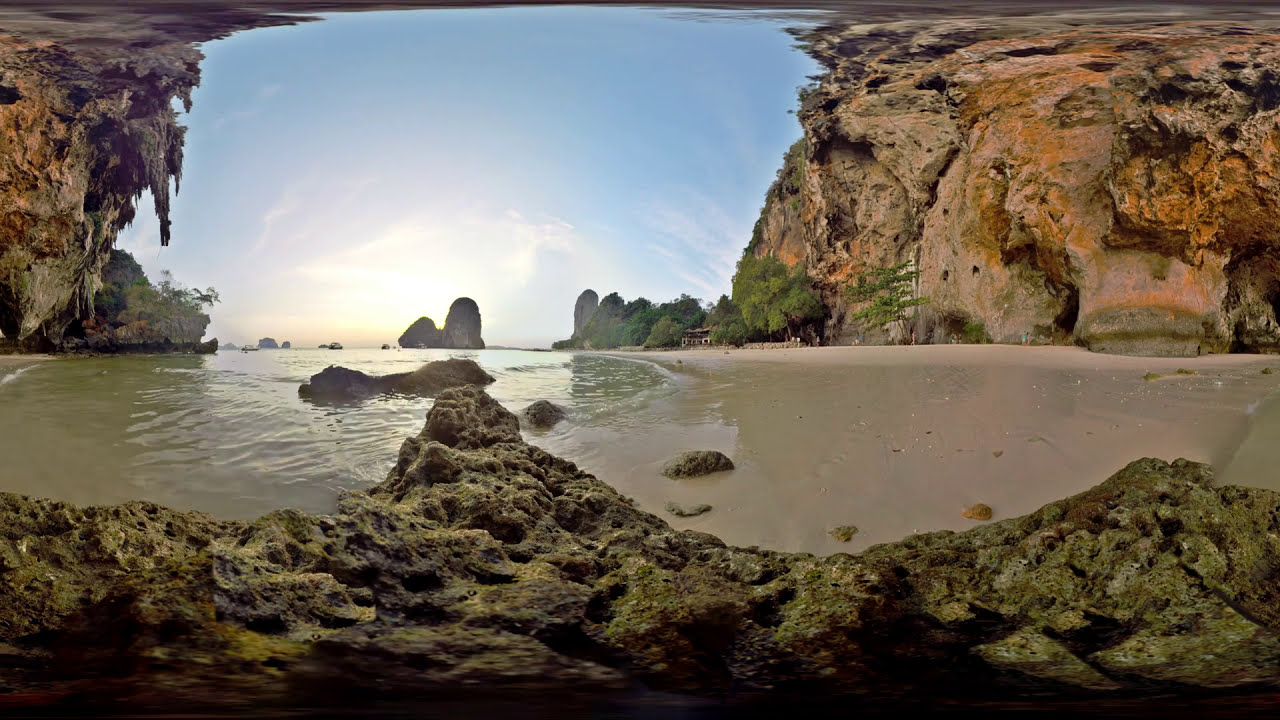This image, appearing like a computer-generated visualization, captures a scenic cove that resembles a tropical beach locale you might find in the Southern Philippines, Thailand, or parts of Vietnam. Horizontally aligned and rectangular, the photo is framed by textured cliff sides on the top, left, and right. These cliffs are a blend of brown, gray, orange, and green hues, richly detailed with their rocky surfaces embellishing the sides of the image. The blue sky above is adorned with wispy, white feather-like clouds, indicating a serene, possibly pre-sunset atmosphere.

In the middle of the frame lies a body of still, muddy-brown water, flat with no waves, suggesting it might be a lake or an inlet. Notable are the gentle ripples on the left side, surrounding a small rocky protrusion. The scene evokes a sense of quiet, accentuated by the foreground's strip of rock extending from left to right. This rock is heavily textured with browns and greens, coated with patches of moss, enhancing the natural, untouched feel of the landscape. Despite resembling a natural setting, there are suggestions of a synthetic or digitally altered appearance, marred slightly by distortions that mimic the interlaced feedback of an old VHS tape.